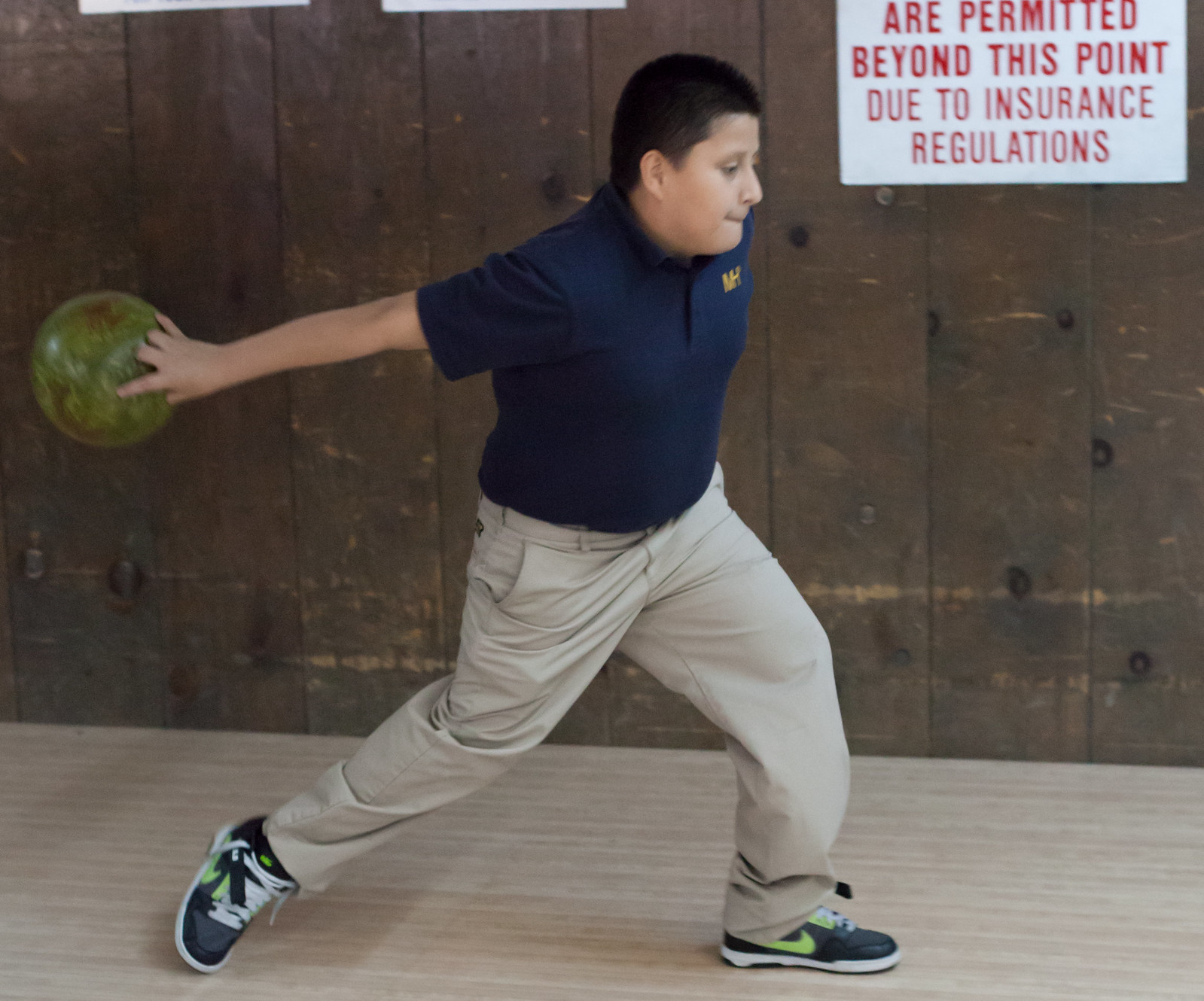The image captures a middle school-aged boy, likely around 12 years old, in the midst of a bowling motion. He is wearing a blue polo shirt adorned with a gold "MH" emblem near the pocket area, and a pair of tan khaki pants. His short black hair complements his casual yet focused demeanor. A green and brown bowling ball is held in his hand behind him, indicating he's poised to release it. His stance is dynamic, with one leg lunged forward and the other kicked back, emphasizing his readiness. He sports gray Nike tennis shoes with green emblems and white laces. The background consists of vertical wooden planks, alongside a rectangular white sign with red lettering that reads, "are permitted beyond this point due to insurance regulations." The light tan hardwood floor completes the setting of this moment in a bowling alley.